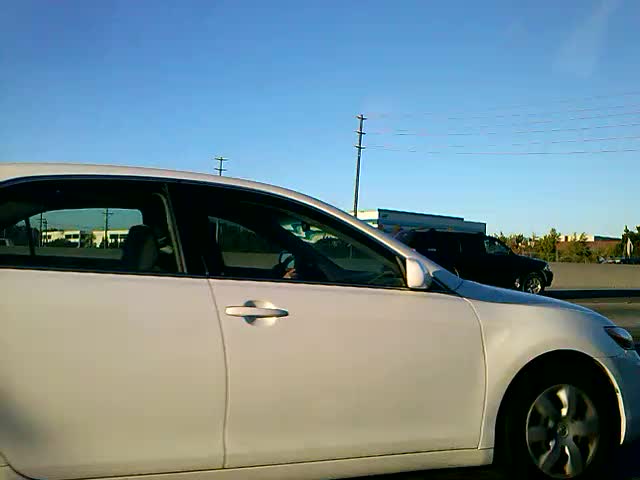The image depicts a first-person perspective of a moving white sedan, with a visible pair of hands gripping the steering wheel inside. The photograph is taken from an angle facing the passenger side door. The car appears to be in motion, evidenced by the slight blur on its tires and rims. In the background, slightly above the hood and to the right of the white sedan's windshield, is a blue SUV. A short gray wall extends horizontally behind the SUV, framing the mid-ground of the image. Beyond the wall, a clear blue sky with few clouds is visible, along with power lines that extend into the distance on the right side of the image. Scattered behind the white sedan and its surrounding area are buildings, some with a blue and white facade, and a cluster of trees on the right. The scene is well-lit, suggesting daytime, and captures a moment of urban activity.